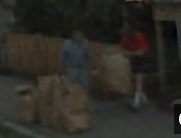This small, rectangular photograph, measuring approximately one inch by an inch and a quarter, depicts a scene that appears quite dark and somewhat obscure. In the center of the image, a man is visible, dressed in a blue shirt and blue pants. To the right of him stands a woman wearing a red shirt that appears to end at her elbows, paired with a black skirt and white, almost knee-high socks. In the foreground and also positioned next to the woman but behind the man, there are several large beige-brown objects resembling oversized bags, standing nearly as tall as the man's legs and reaching about two-thirds the height of the woman. The background of the photograph is entirely black, adding to the overall indistinctness of the scene. Additionally, to the right of the woman, there is what appears to be an open doorway. The image's darkness and lack of clarity make it challenging to discern finer details.